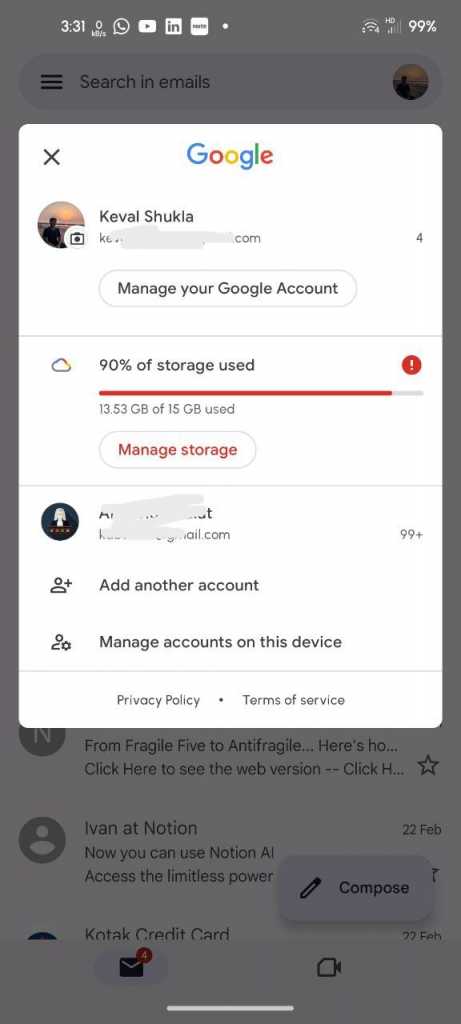This is a detailed screenshot caption of a mobile phone screen displaying the Google account management interface, with the battery level at 99% charged. The interface includes a search bar with the placeholder text "Search in emails" set against a gray background. At the top of the screen, a white box prominently displays the text "Google."

Below this, the account summary shows the name Keevil Shukla alongside an obscured email address. A button labeled "Manage your Google Account" is positioned underneath. The storage usage section follows, indicating that 90% of the storage is used (13.53 GB of the available 15 GB), accompanied by a "Manage Storage" clickable button.

Further down, an icon of a person with an option to "Add another account" is displayed. Next to it, another person icon with a small round circle on the shoulder offers the "Manage accounts on this device" option. At the bottom of the interface, hyperlinks to the "Privacy Policy" and "Terms of Service" are provided. The interface is clean and aimed at facilitating easy navigation and management of Google account settings.